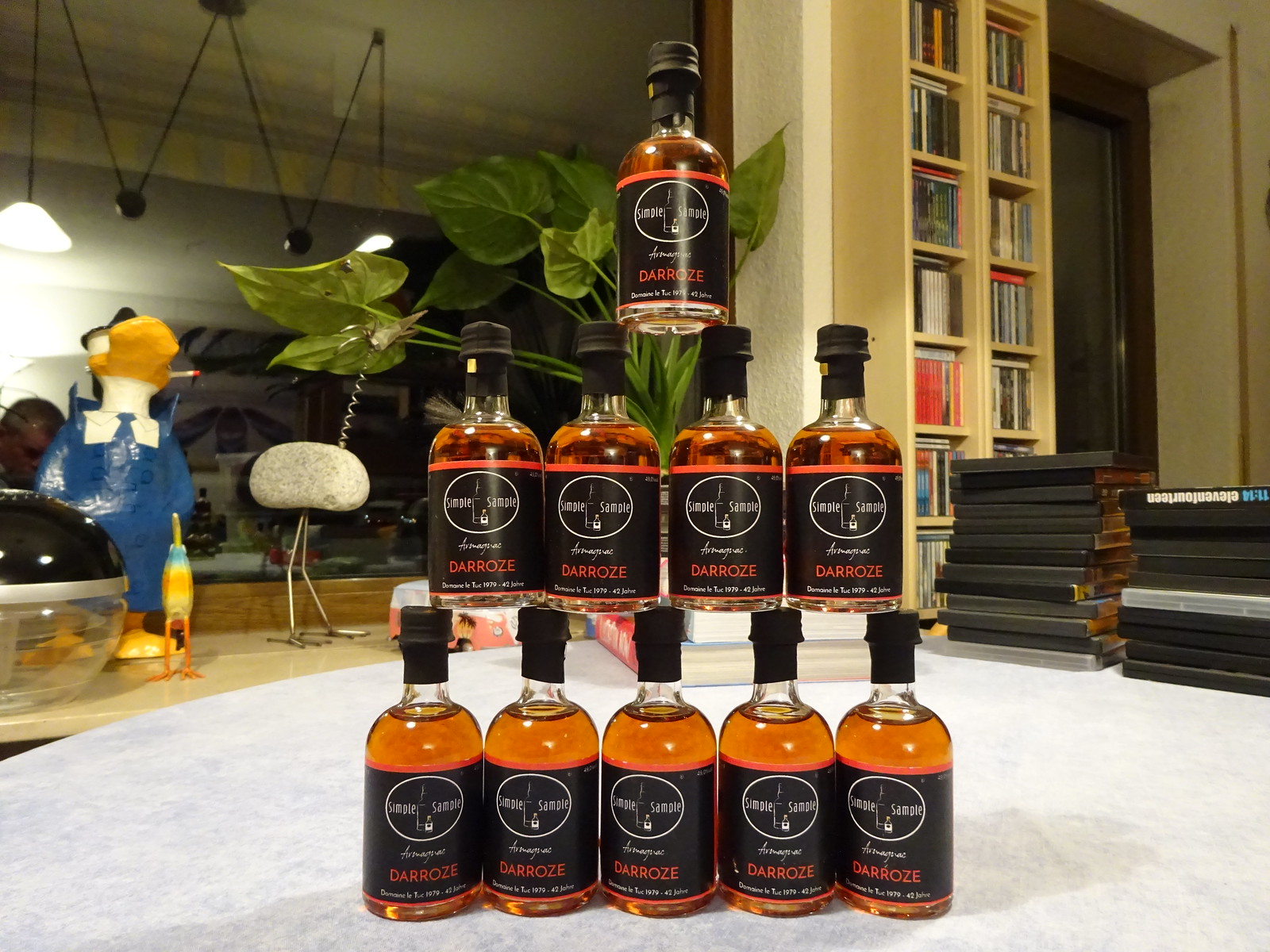This close-up photograph showcases a neatly arranged display of 10 small sample bottles of DeRose liquor. Each bottle features a black label with "DeRose" written in red letters and a white oval circle marked "sample." The bottles, containing a golden-colored liquid, are made of plastic and have black lids. They are expertly stacked in a pyramid formation: five bottles form the base, with four bottles stacked directly above them, and a single bottle perched at the top. This display sits on a white table, possibly in a living area that includes a mix of decor items. To the right of the bottles, there's a stack of DVD covers, and to the left, a porcelain figurine resembling a headless duck in a blue suit is visible. Additionally, a potted plant is placed behind the bottle pyramid, contributing a touch of greenery. In the left background, there is a tall white bookshelf filled with books or DVDs, lending a homely atmosphere to the setting.